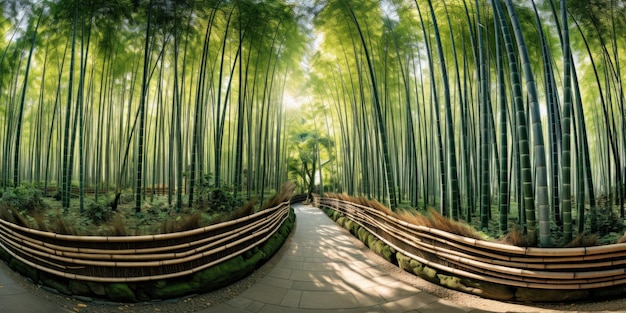The image depicts a peaceful, picturesque bamboo forest scene, with a rectangular stone-paved pathway stretching down the center. The light gray pavers create a steady rhythm leading the eye through the enchanting landscape. On either side of the path, there is a curving bamboo fence made from dried, light yellow bamboo. Inside this fencing stands a forest of tall bamboo plants, their slender trunks stripped of leaves up to about three-quarters of their height, creating an almost surreal, fairytale-like aesthetic. The bamboo trees vary in size and shades of green, with their leafy canopies high above, allowing glimpses of blue sky to shine through. The sun casts intricate shadows on the pathway, adding to the serene ambiance. This scene, with its uncanny yet beautiful charm, could easily be imagined as a perfect bike lane or a tranquil walking path within a wooded park, inviting explorers to venture deeper into its almost otherworldly setting.